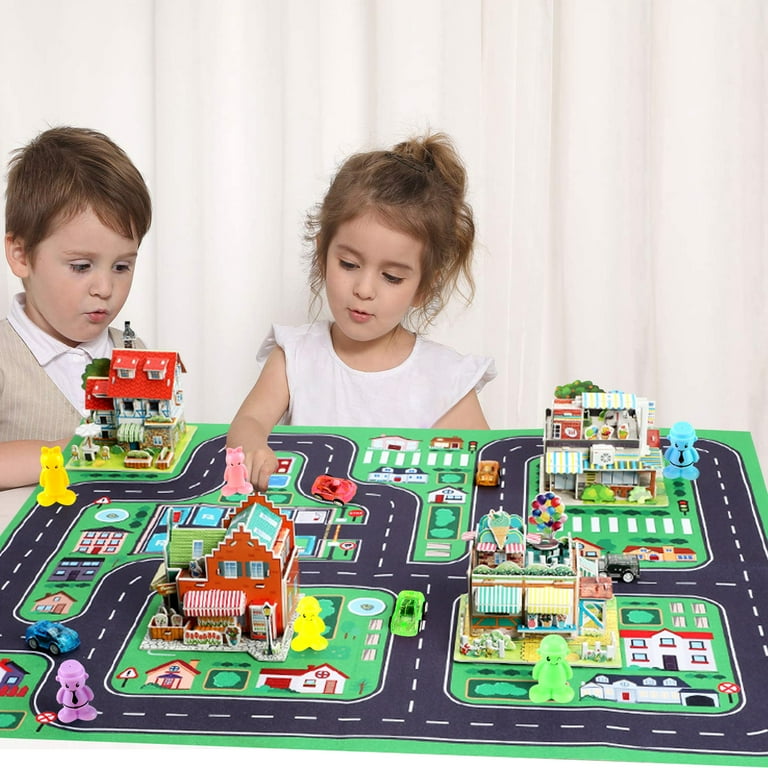In the photograph, two young children—both with brown hair—are engrossed in play in front of rippled white drapes. The boy, positioned on the left, is dressed in a white collared shirt with a beige vest, while the girl in the middle is wearing a sleeveless white dress with her hair styled in a messy bun. They stand behind a vibrant play mat that depicts a miniature city, complete with a winding black road marked by white lines. The mat is dotted with various 3D buildings like houses, barn-like structures, and an ice cream shop. Scattered across this miniature town are colorful toy figurines—purple, green, yellow, and pink—as well as toy cars in an array of hues like blue, green, purple, and orange. The girl is focused on a pink figurine, while the boy engages with a building adjacent to a yellow figure standing on the road. The intricately detailed play mat offers an assortment of buildings and roads, allowing the children to immerse themselves in imaginative play.